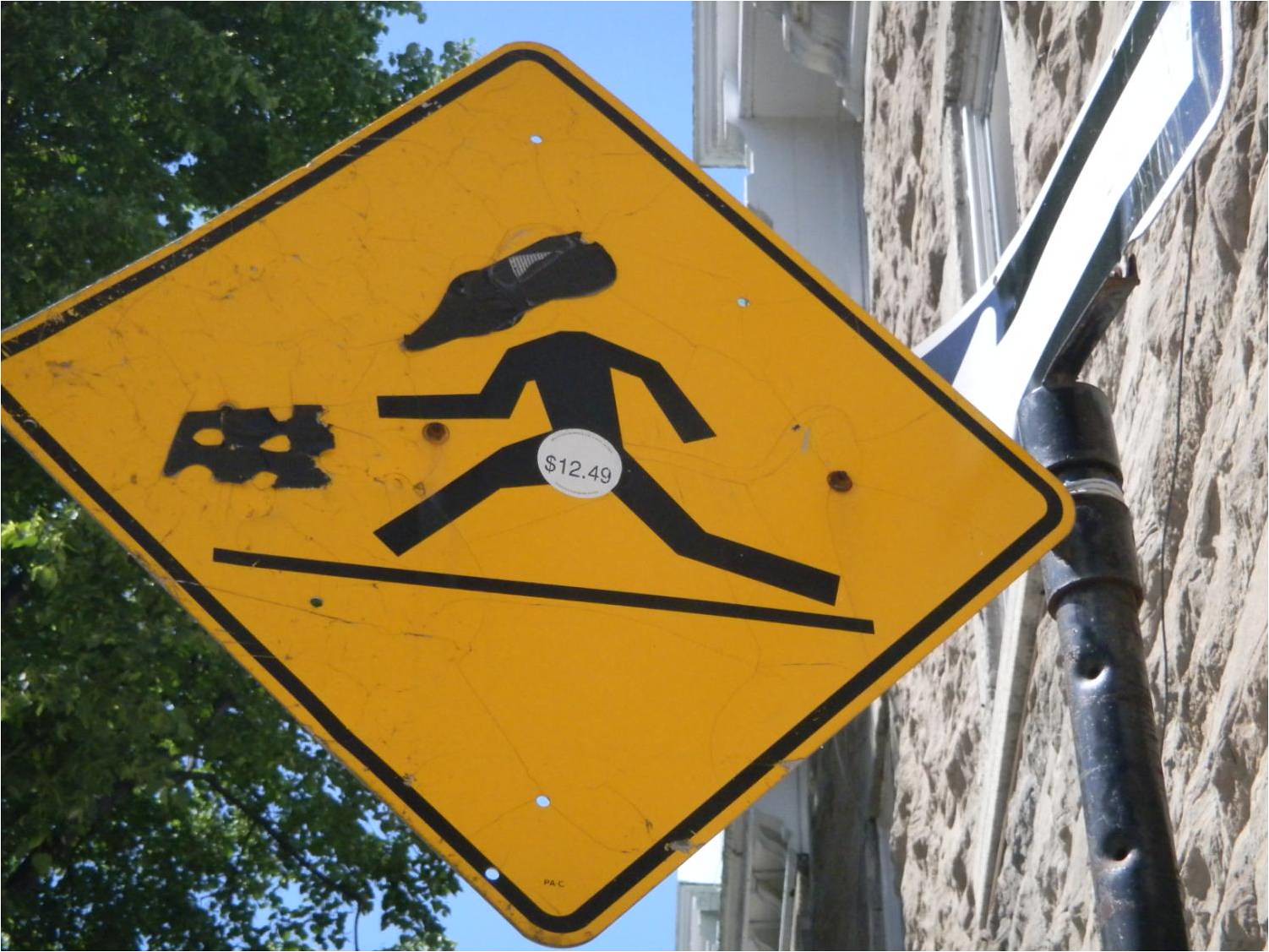The photograph captures a vandalized pedestrian walking traffic sign situated on the side of a street. The sign is a bright yellow diamond shape with black writing and depicts a running figure, whose head has been altered to resemble that of a mouse. Below the figure is a black line, making it appear as if the character is running. A white circular sticker in the middle of the sign declares a price of $12.49 in black text. To the right of the sign stands a light gray or white brick building, accompanied by a black pole supporting a white arrow on a black background. The scene is framed by a clear light blue sky and, on the far left, a green tree. Additionally, someone has drawn an object with two holes to the left of the figure on the sign.